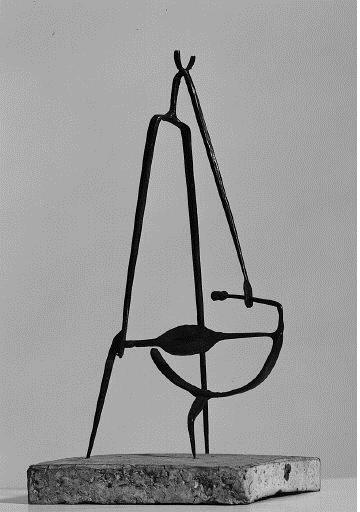The image features an abstract black metal sculpture set atop a thin granite or cement square base, appearing similar to a sidewalk tile. The sculpture comprises a complex arrangement of thin, welded or twisted metal rods forming various shapes and lines. At the top, a prominent horseshoe-like form points upward, resembling the letter "U," from which a line descends. Below, two parallel lines create a leg-like structure, and another curved piece extends from the bottom, curling upwards and then back down. The sculpture is characterized by its intricate, open-to-interpretation design, with elements that loop and weave in multiple directions, creating a dynamic, yet somewhat shapeless appearance. The entire composition rests against a gray background, emphasizing the stark contrast of the black metal sculpture against its subtle surroundings.